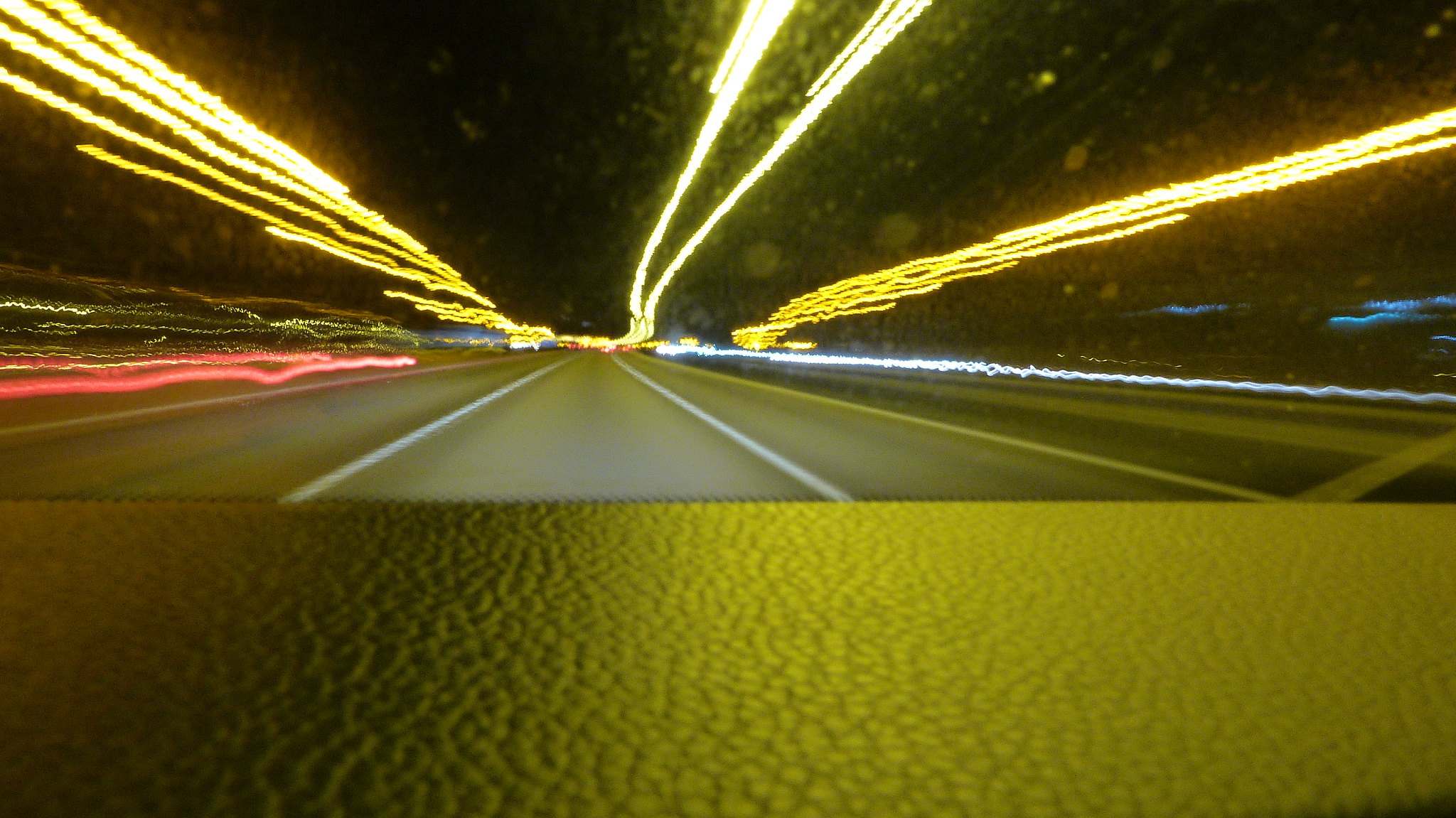The image is a vivid night-time photograph taken from the front windshield of a speeding car. The shot captures the top of the dashboard, which appears to be leather, closely pressed against the glass. The road extends straight ahead into the horizon, divided into lanes marked by white lines. The motion blur from the car's speed creates an array of vibrant, streaky lights arching across the pitch-black sky. Fluorescent streaks of yellow, white, blue, and pink, likely from streetlights and buildings, blend together, giving the impression of light speeding towards the horizon. Red taillights from another vehicle appear off to the left-hand side, adding to the dynamic and fast-paced feel of the scene. The combination of motion blur and colorful light trails makes the photo a captivating depiction of high-speed travel at night.